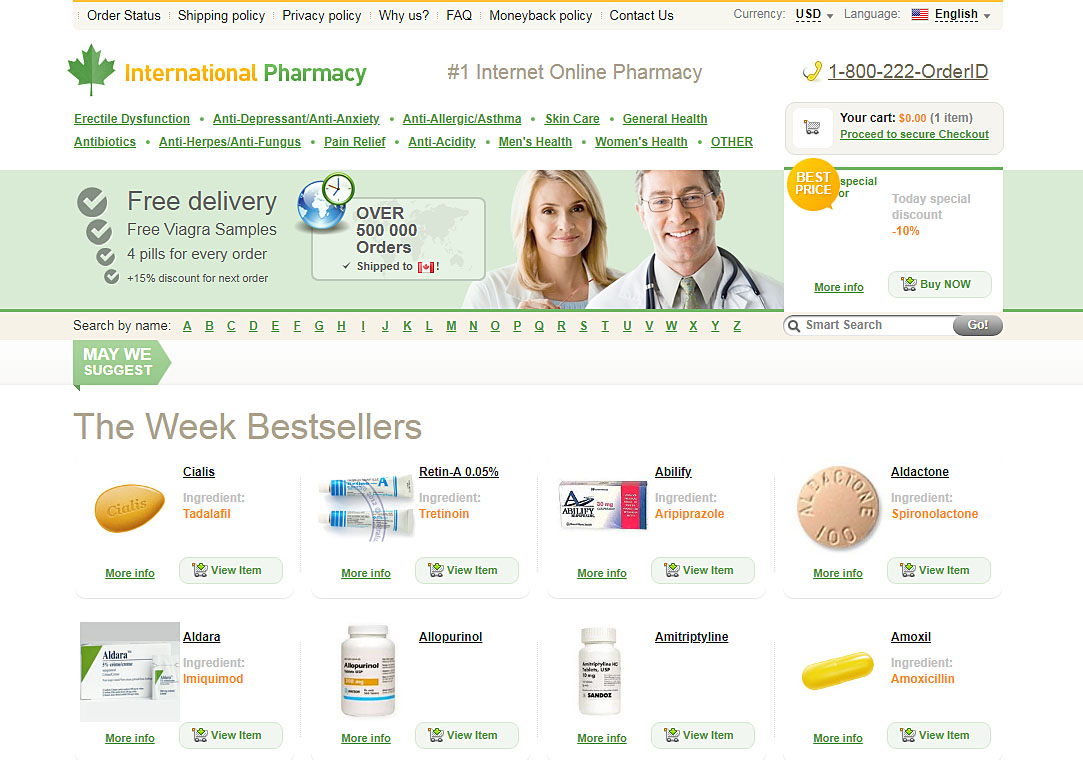A screenshot of the International Pharmacy website presents a detailed and organized layout, emphasizing its status as the "Number One Internet Online Pharmacy." The website prominently displays the contact number 1-800-222-ORDER-ID for easy customer service access. The top menu includes essential navigational links: Order Status, Shipping Policy, Privacy Policy, Why Us, FAQ, Money Back Policy, and Contact Us. Users have the functionality to set their preferred currency and language, with the current settings showing USD and English.

Below the logo, various popular categories are listed, such as Erectile Dysfunction, Antidepressant/Anti-Anxiety, Anti-Allergic/Asthma, Skincare, General Health, Antibiotics, Anti-Herpes/Anti-Fungus, Pain Relief, Anti-Acidity, Men's Health, Women's Health, and Others. 

A prominent banner featuring a doctor and a nurse highlights special offers like free delivery, complimentary Viagra samples (four pills per order), a 15% discount on the next order, and a note boasting over 500,000 shipments to Canada. The site facilitates easy drug searches with a "Search by Name" section displaying clickable alphabet letters and a "Smart Search" feature with a go button.

At the bottom, a "May We Suggest" section showcases this week's bestsellers, arranged in two rows with four items each, featuring popular medications such as Cialis, Retin-A, and Abilify. The clean organization and comprehensive details serve to attract and inform potential customers effectively.